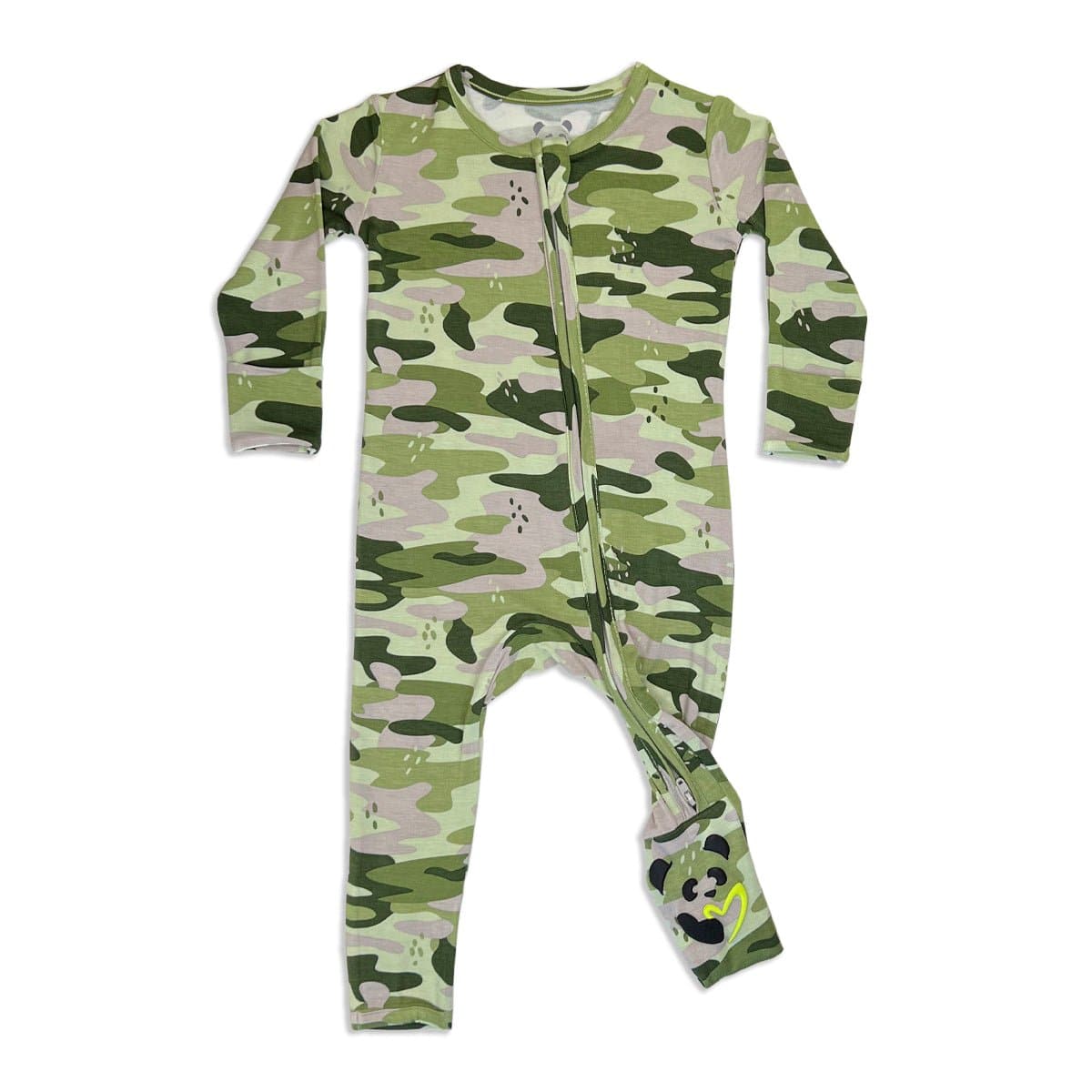The image showcases a detailed, camouflage-patterned onesie primarily in various shades of green, ranging from olive to dark forest green, along with occasional beige and hints of a pinkish-purple hue. Designed for a toddler or young male child, the onesie features a standard collar and mid-length sleeves that reach the elbows. A prominent zipper runs from the neck down to the right leg of the garment. On the right leg, there is an illustrative detail of a panda bear. This panda bear has black eyes, nose, ears, and one black arm, and it is depicted holding a fluorescent lime green heart. The overall aesthetic combines a rugged military camouflage with a playful panda bear element.